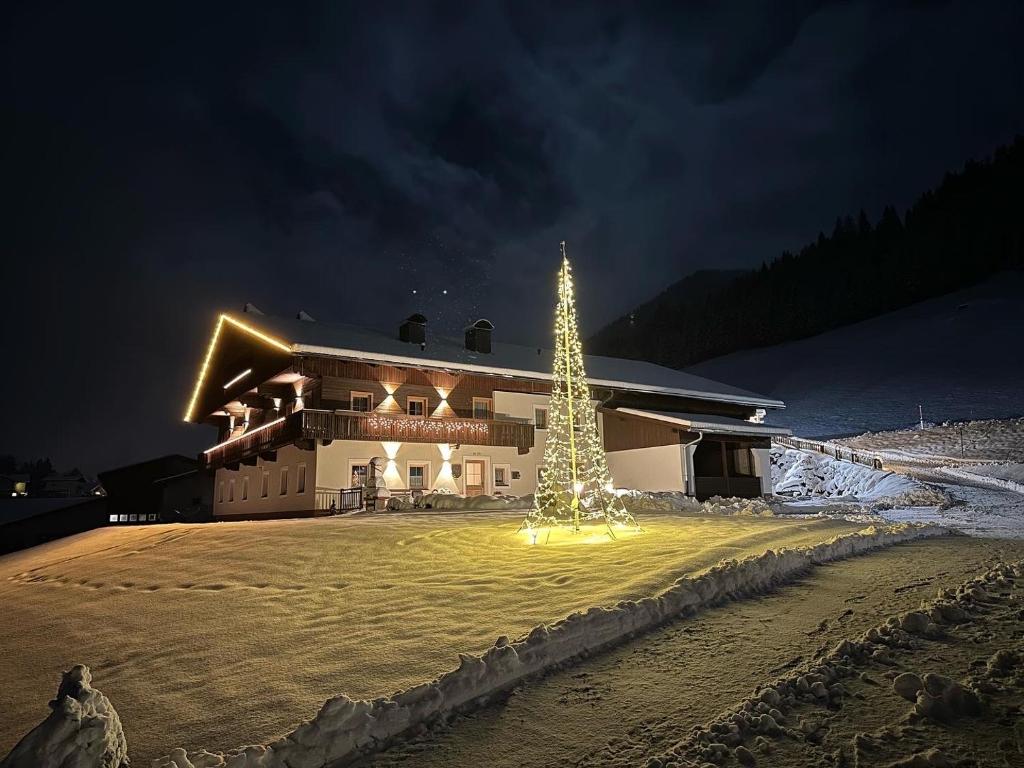The photograph captures a serene and festive nighttime scene outside a two-story house, showcasing a winter wonderland covered in thick snow. The house itself features a dark brown wooden upper story and a white lower story, complete with a wrap-around deck on the upper level and numerous windows on both floors. Illuminated Christmas lights adorn the house, outlining the A-frame of the roof, draping over the banisters, and accentuating the home's front and side profiles. 

In the front yard, a striking artificial Christmas tree made entirely of lights, predominantly white but featuring other colors, stands tall, emitting a warm glow that enhances the festive ambiance. The tree's lights are meticulously wrapped around a central pole to form the traditional conical shape. Footprints pepper the otherwise smooth snow, showing signs of activity, while the driveway and sidewalk appear to have been recently shoveled and plowed, creating clear paths through the snow.

All of this is set against a backdrop of a very dark, almost black sky, with a few indigo-hued clouds faintly visible but no stars to be seen. Further enhancing the picturesque setting, there is a tall hill behind the house with trees poking out, making the scenery both magnificent and tranquil. The overall effect is a cozy, inviting home radiating holiday cheer amidst a peaceful, snowy landscape.